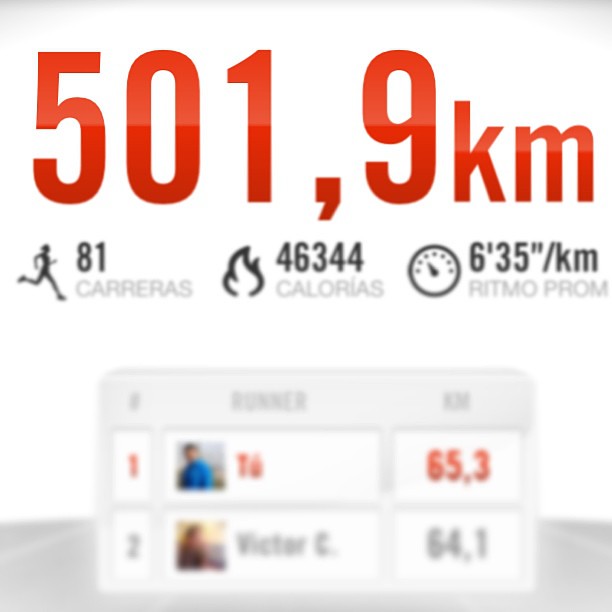The image appears to be a screenshot from a Spanish-language running app or exercise equipment readout, set on a white background with slight gray borders at the top and bottom. Dominating the top of the image, in large red text, is "501,9 KM" indicating a distance of 501.9 kilometers. Below this, the screen is divided into several readouts. 

First, there is a black silhouette of a person running next to the number "81" and the label "Carreras," which means races. Following that is a black flame icon beside "46,344 Calorias," indicating the number of calories burned. The third readout features a black speedometer icon accompanied by the time "6'35"/KM" and the label "Ritmo Prom," likely referring to an average pace of 6 minutes and 35 seconds per kilometer.

At the bottom, a blurred-out leaderboard showcases two users’ results. The first user, highlighted in red, is number one with "65,3 KM," and the second user, in gray, identified as "Victor E," has "64,1 KM." Both user icons are too blurred to make out the details clearly.